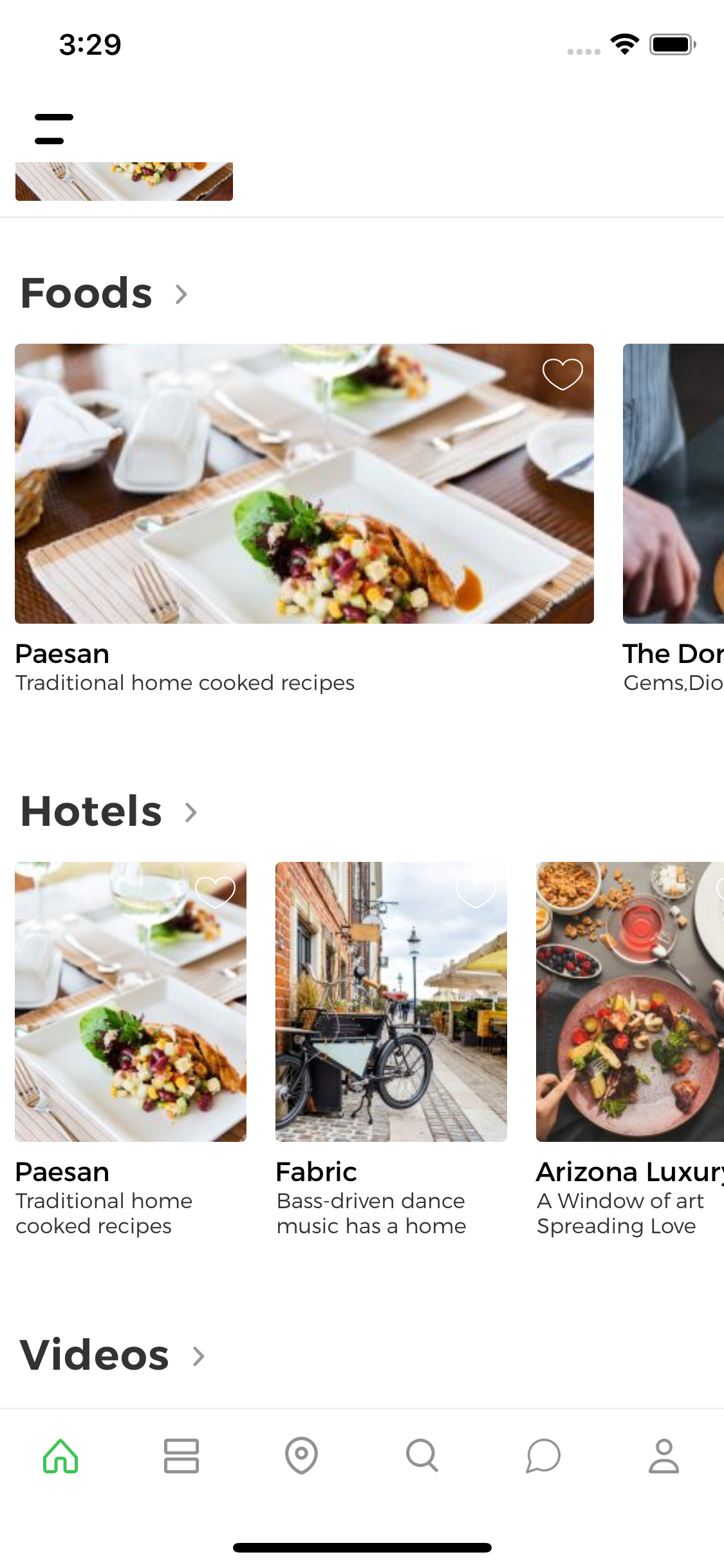The image displays a cell phone screen in detail. The top left corner shows the time "3:21," while the top right corner indicates a full Wi-Fi signal and a fully charged battery icon. Below these icons, there's a hamburger menu represented by two horizontal lines, which seems unusual. 

Beneath this, a partially visible image can be seen, followed by the bold text "Foods." Below "Foods," there's an image of some food accompanied by a label that reads "PAESAN traditional home-cooked recipes." To the right of this, another partial image and partial text is visible, with one word being "the." 

Further down, the bold text "Hotels" in black writing appears. Below this section, there are three images. The first image is identical to the "PAESAN traditional home-cooked recipes" picture previously mentioned. 

In the center, there's an image of fabric with a bicycle or similar object hanging above a street, captioned "Bass driven dance music has a home." On the far right, another image is labeled "Arizona luxury: a window of art, spreading love" and displays a plate of food, a drink, and additional food items.

At the bottom of the screen, a label reads "Videos." The very bottom of the cell phone screen features an array of icons: a home button, a hamburger menu button, a location pin button, a search button, a chat bubble button, and a person icon.